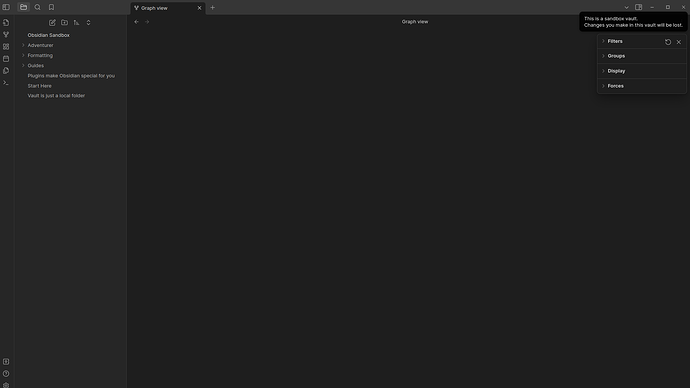The image depicts a low-resolution interface of an application that mimics the tabbed layout commonly found in web browsers, but it is not a browser. The primary background color of the interface is a very dark gray. 

On the far left, there is a vertical column featuring several menu options in white text, though the text is unreadable due to the low resolution. Adjacent to this column, still on the left side but slightly further right, is another vertical row containing small, indistinct icons aligned from top to bottom.

At the top of the interface, there is a tab labeled "Graph View," difficult to discern but identifiable, with a small "X" button for closing the tab next to it. To the right of this tab, there is a clearly visible white "+" button, presumably for opening a new tab in the application.

In the top-right corner, familiar Windows control icons for close, maximize, and minimize are present. Next to these are two additional, illegible white icons. Beneath these icons, extending across the top, is a black banner with some text in the upper left-hand corner, which is also unreadable at this resolution. Below this banner, there are four menu options displayed in white text that are similarly illegible.